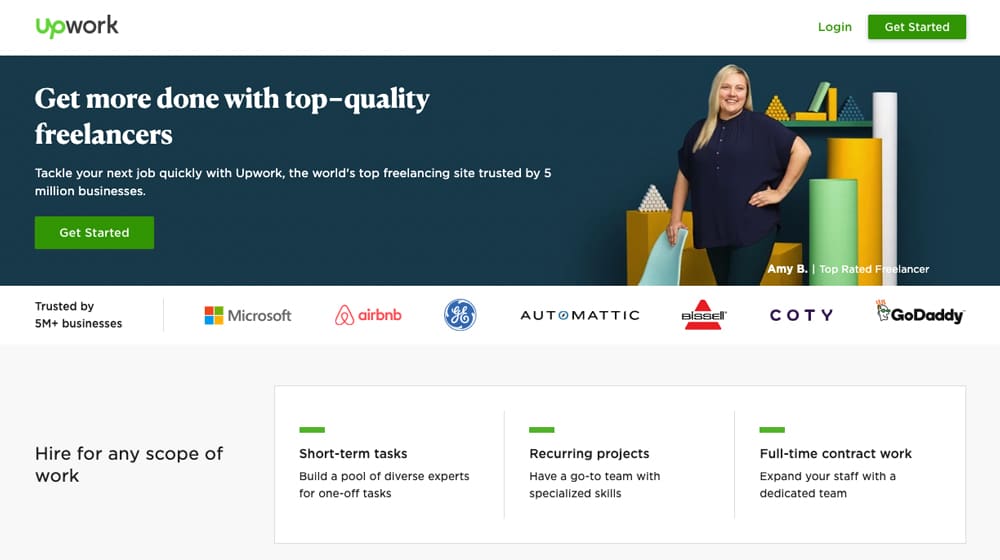This horizontal rectangular image prominently features brand messaging from Upwork, a popular freelancing platform. 

In the upper left corner, the word "Up" in green text is followed by "work" in black lowercase letters. To the right, the words "Login" in green text precede a green horizontal rectangle that reads "Get Started" in white font.

The largest area of the image, which is blue-green, carries an inspiring message in white text on the left: "Get more done with quality freelancers." Below this, smaller white text reads, "Tackle your next job quickly with Upwork, the world's top freelancing site trusted by 5 million businesses."

Farther down the image, there's another green horizontal rectangle with the words "Get Started" in white. To the right of this box is a picture of a woman wearing a blue shirt and dark pants. Her left hand rests on a light-colored chair back, while her right hand is on her hip. Nearby, several foam rollers in green, orange, and white colors are visible, along with other geometric shapes on a shelf behind her.

Beneath the image, in black font, it states, "Trusted by 5M+ businesses," followed by the logos of various companies: Microsoft, Airbnb, GE, Automatic, Cody, and GoDaddy.

The bottom section of the image highlights Upwork's versatile hiring options, with three horizontal rectangular boxes, each with a short green line above the text:
- "Short-term tasks: Build a pool of diverse experts for one-off tasks."
- "Recurring projects: Have a go-to team with specialized skills."
- "Full-time contract work: Expand your staff with a dedicated team."

This detailed layout clearly communicates the benefits and versatility of using Upwork for various business needs.